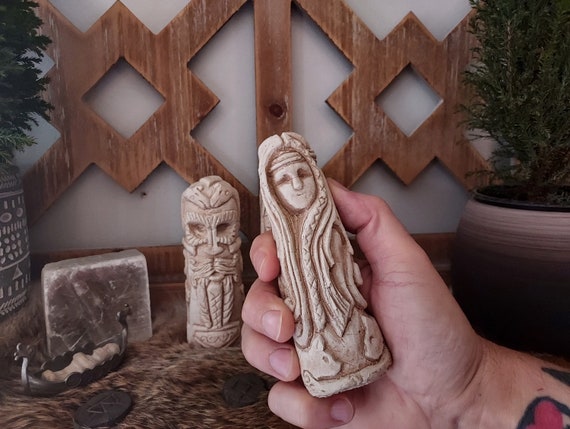The image depicts an intricate scene brimming with historical ambiance. Central to the composition are two exquisite marble figurines, skillfully crafted to represent a Viking male and female. One of these figurines is gently grasped by the right hand of an individual whose forearm bears a distinctive tattoo. To the left of the figurines stands a meticulously detailed model of a Viking longship, further emphasizing the Norse theme.

At the bottom of the frame, an array of carved flake stones is arranged, contributing to the ancient and archaeological vibe of the scene. A potted plant with delicately etched designs adds a touch of natural elegance and symmetry on the left side of the image. The background showcases an angular wooden design with a square at its focal point, emanating lines that add depth and complexity to the setting.

The lighting, seemingly originating from the center-left, casts a warm glow across the image, highlighting the textures and enhancing the intricate details of the marble carvings and other elements present.